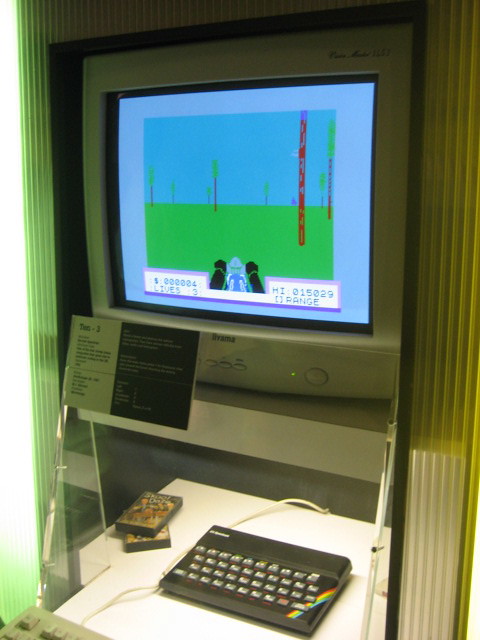In this vertically-oriented photograph, we are presented with a detailed view of a modern office workspace. Central to the composition is a sleek white desk which serves as the focal point. Atop the desk sits a sophisticated keyboard, colored black with silver or gray buttons, contributing to the workspace’s high-tech aesthetics. To the left of the keyboard, two cartridges are neatly positioned, adding to the array of office and gaming paraphernalia. Above the desk is a screen, likely a monitor or television, vividly displaying a video game. The game features a dynamic scene with characters and elements in shades of green, blue, red, and black; prominently visible are two black dogs and a human figure. On the lower left corner of the screen, the game status indicates "Lives: 3," while the lower right corner shows the score as "High: 015029" alongside the word "Range." This detailed glimpse into the workspace captures a blend of productivity and leisure, showcasing the occupant’s dual interest in work and gaming.